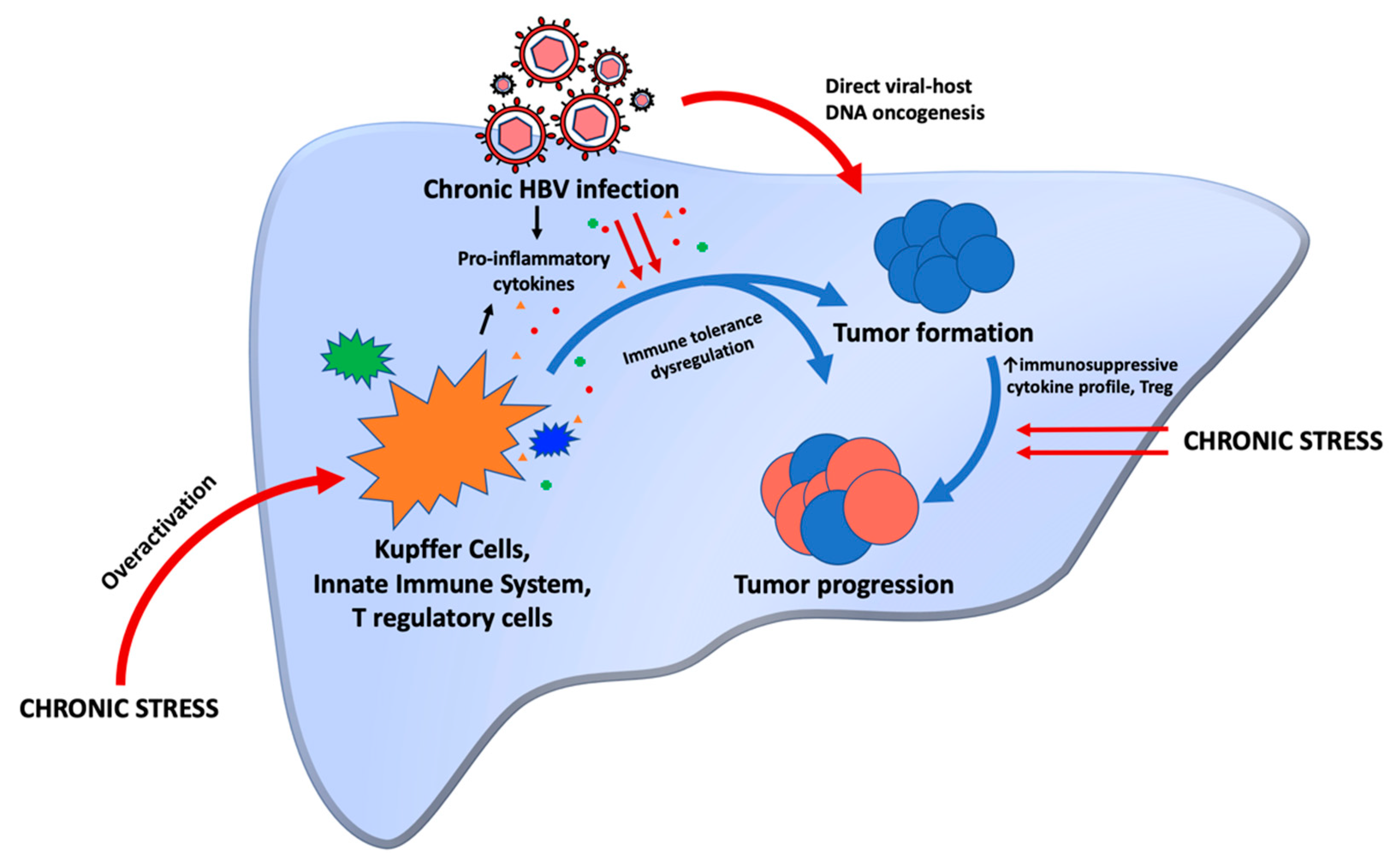The image is a detailed medical diagram displaying the progression of a tumor under chronic stress and chronic HBV infection. The diagram is primarily set on a free-form blue blob, resembling a water puddle. In the bottom left corner, a red arrow labeled "chronic stress over-activation" points to a starburst graphic, evocative of a comic book explosion. Various colored shapes within the starburst represent "Kupffer cells," "innate immune system," and "T-regulatory cells."

Adjacent to this, hexagonal shapes surrounded by a viral shell mark "chronic HBV infection," with connecting arrows highlighting "pro-inflammatory cytokines." The blue double-split arrow extends from this cluster, indicating "immune tolerance and dysregulation." Another arrow from the HBV cluster leads to "direct viral host DNA oncogenesis," shown with a group of spheres labeled "tumor formation."

Further along, additional indicators of "immunosuppressive cytokine profile" and "Treg" cells continue from the tumor formation graphic. The final arrow from the tumor formation scene shows larger blue and orange spheres, symbolizing "tumor progression."

The top section of this diagram ties together the key processes starting with overactivation and cellular responses, moving through viral infection impacts, to the core progression from initial tumor formation to advanced stages heavily influenced by chronic stress factors.